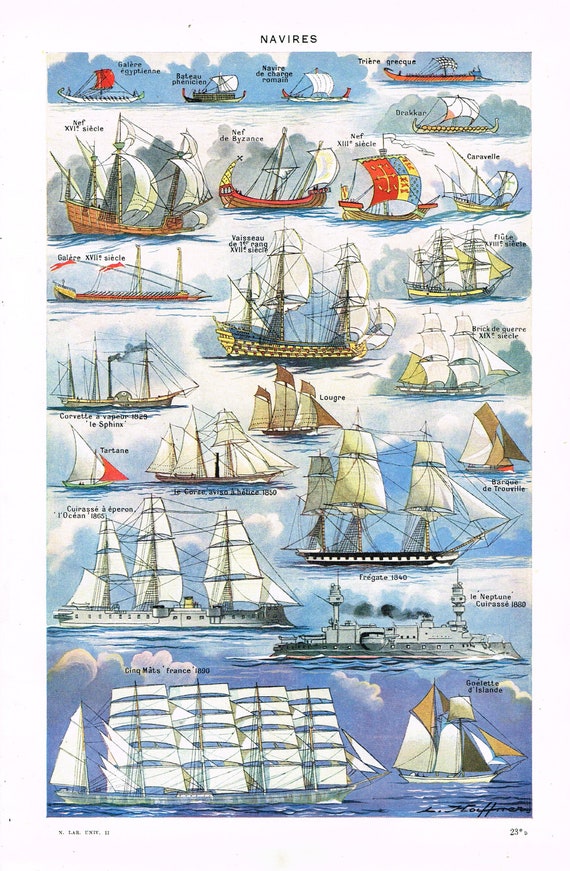The image is a detailed, vertically-oriented diagram featuring approximately 15 historically significant sailing vessels, captioned in French. The diagram, scanned from a book, begins with older vessels at the top, progressing to modern ships at the bottom. The title at the top of the page reads "NAVires," showcasing a range of boats from different eras. The top row includes ancient vessels like an Egyptian gallery, a Phoenician boat, a Roman army boat, and a Greek trireme. Following these are a drakar, labeled "D-R-A-K-K-A-R," as well as larger sailing ships with multiple white sails, some adorned with heraldic symbols.

As the illustration continues, mid-19th century tall ships appear, characterized by multiple masts and sails typical of the 1800s. Below these are frigates and cuirasses, with a transition to more modern naval vessels. Notably, towards the bottom is a gray, metallic ship devoid of sails, featuring a smokestack emitting smoke. The final vessel at the bottom is a five-masted ship. The background colors transition from blue skies and clear water at the top to more diverse hues towards the bottom, enhancing the historical progression of the ships depicted. Each vessel is meticulously labeled in French, with artist attribution to L. Hoffman and a notation at the bottom right reading "NLAB UNIV 23."